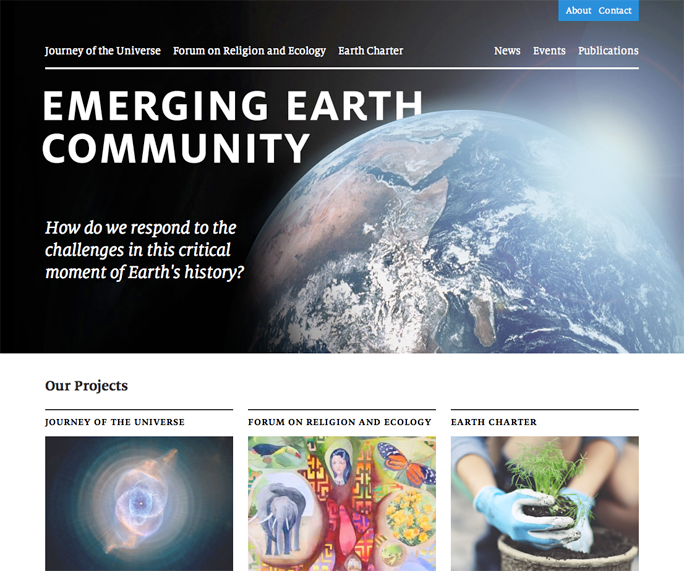Screenshot of the "Emerging Earth Community" homepage. The largest text on the page, "Emerging Earth Community," is prominently displayed in large white capital letters towards the upper left. Behind this title is a captivating zoomed-out image of Earth from space, surrounded by the vastness of the black cosmos. At the top of this section, smaller white text reads, "Journey of the Universe, Forum on Religion and Ecology, and Earth Charter." 

Adjacent to this, the white text continues with "News, Events, and Publications." Towards the upper portion of the site is a lighter blue box containing the words "About" and "Content." Beneath the main title, "Emerging Earth Community," a subtitle in smaller white text poses the question: "How Do We Respond to the Challenges in This Critical Moment of Earth's History?" Directly below this section is a box with a white background containing the header "Our Projects" in black text.

The content of the page is organized in three horizontal sections, each featuring a unique image related to their respective projects:
1. The first box displays another image of space with the black text above it reading "Journey of the Universe."
2. The middle box shows what appears to be a praying woman, an elephant, and a butterfly, with "Forum on Religion and Ecology" written in black text above it.
3. The last box contains an image of a person planting something in a planter while wearing blue gloves, with the text "Earth Charter" positioned above it.